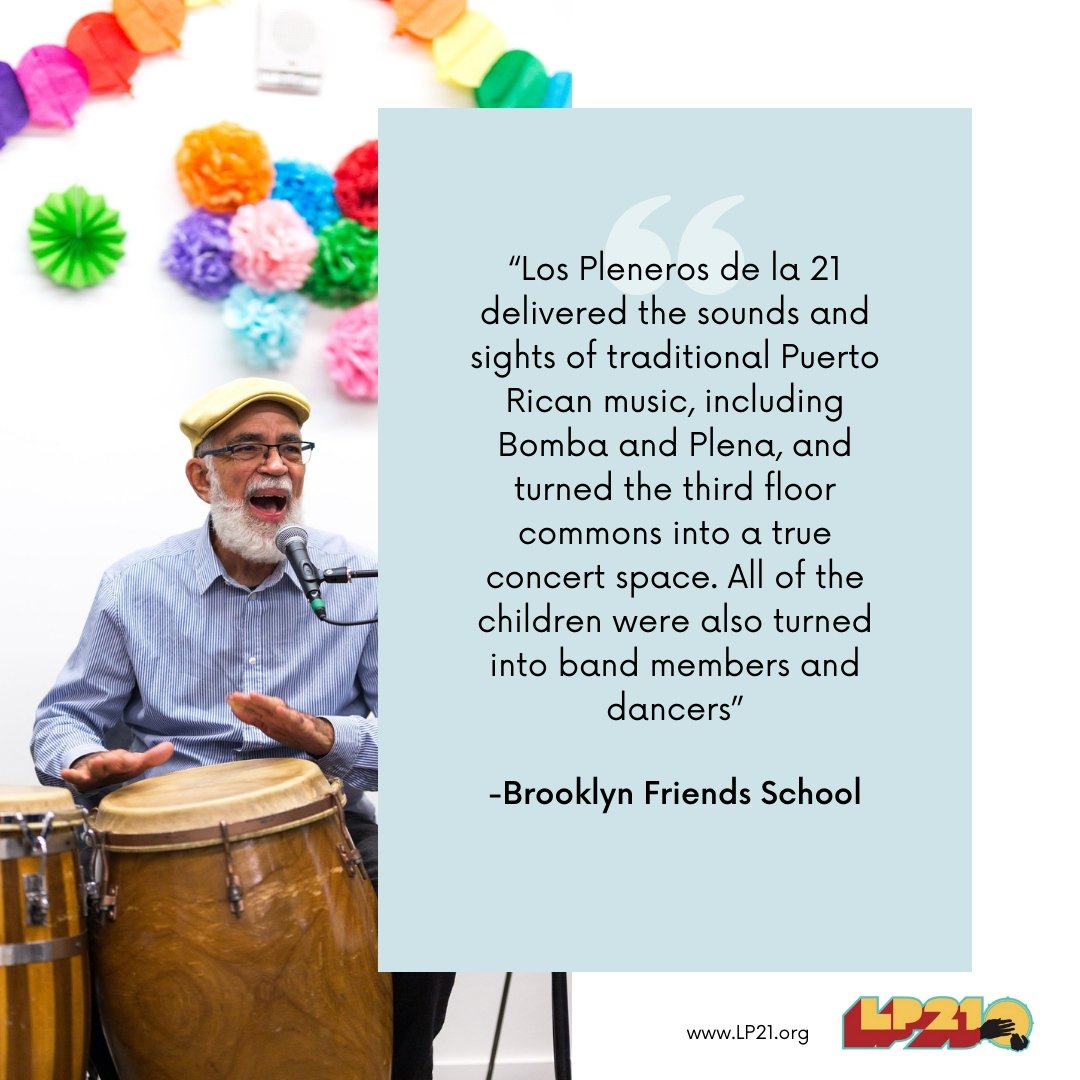This vibrant photograph captures an older man passionately playing bongo drums against a meticulously decorated white wall, possibly during a festive celebration or birthday party. The man, dressed in a blue shirt, yellow cap, and glasses, sports a white beard and seems absorbed in his performance. The bongo drums he is playing have wooden bodies with light brown drumheads, lending an authentic touch to the traditional Puerto Rican music scene.

The backdrop is a cascade of colorful decorations, featuring pink, orange, purple, and bright blue, comprised of pom-poms and paper flowers, creating a cheerful and inviting ambiance. A string of decorations and a banner enhance the festive feeling, while a significant portion of the wall space is dominated by a large blue text box.

The text within the box reads: "Las Planos de la 21 deliver the sounds and sights of traditional Puerto Rican music including bamba and plena, turning the third floor commons into a true concert space. All of the children were also turned into band members and dancers," underscored by the bold text "Brooklyn Field School." Additionally, the web address "www.lp21.org" is displayed, along with a stylized logo of LP 21 in yellow and red.

The setting emphasizes a communal and educational atmosphere, with the Brooklyn Friends School noted for hosting this event. The strategic placement of the man to the left and the textual information to the right balances the photograph, making it both visually appealing and informative.